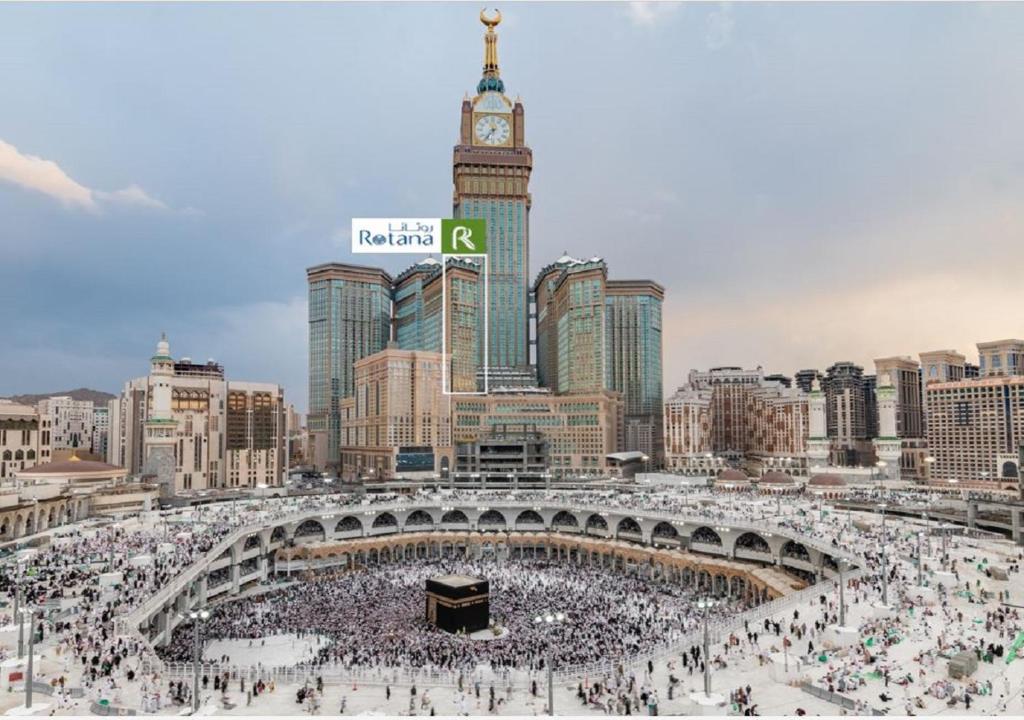The image showcases a bustling cityscape dominated by a prominent skyscraper adorned with a bell tower and a golden spire, marked with the text "ROTANA" on a white square, with the letter R set against a green background. The architecture is modern, featuring many large buildings with numerous windows surrounding the central tower. Below, an expansive area teems with hundreds of people, giving the impression of a densely populated, vibrant hub. This central area resembles a coliseum or a circular city space, with arcs and multiple layers, as well as a distinctive black cube-like structure at its core, suggesting a significant religious site that could be Mecca, with people circumambulating. The sky above transitions from darker blue on the left to lighter blue on the right, with some clouds scattered throughout, creating a dramatic backdrop to the sprawling urban landscape. The ground in the central area appears to be a pristine white, highlighting the contrast between the architectural elements and the crowd of people that fill the scene.